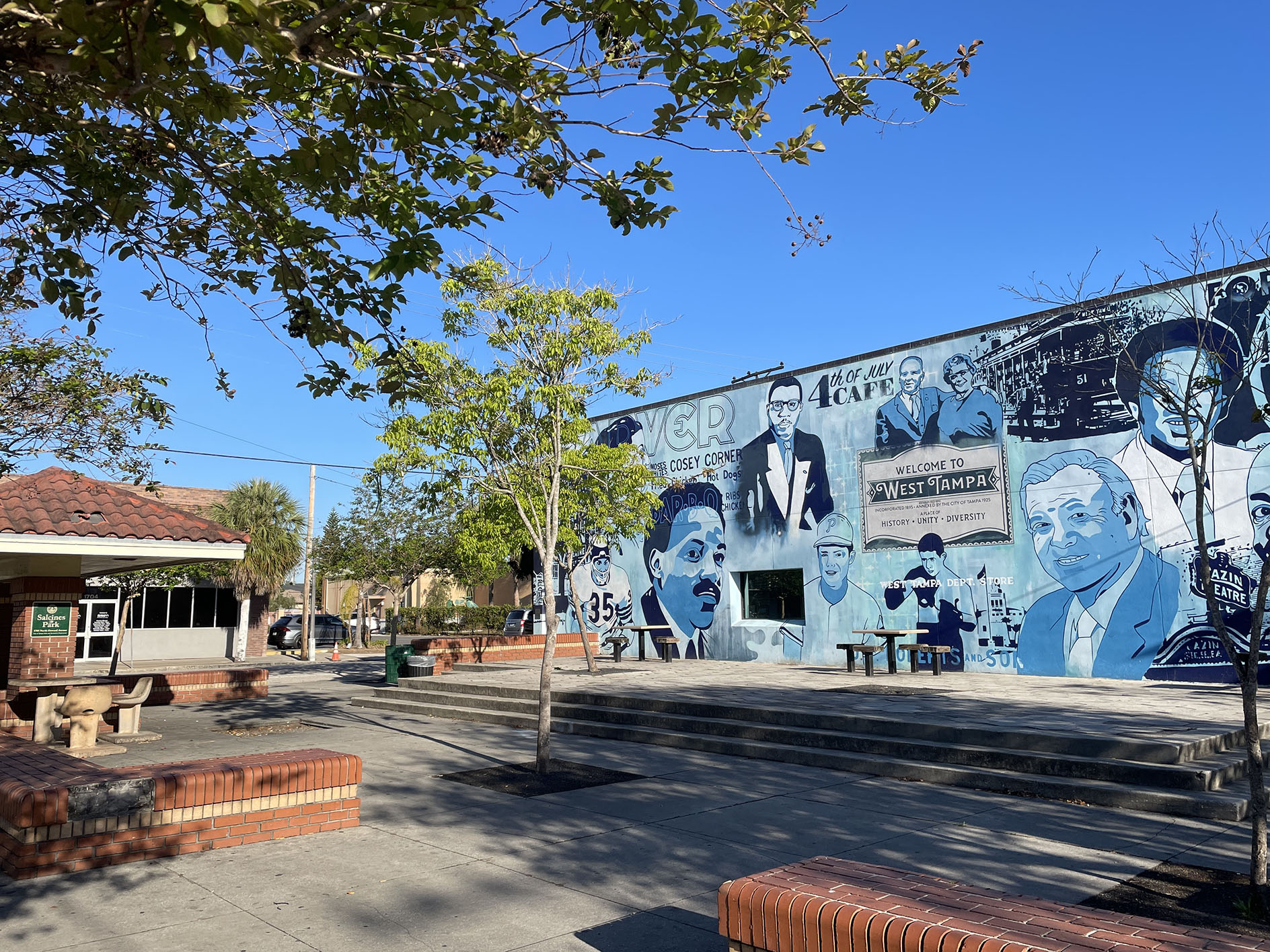The image captures a vibrant small town area dominated by a large, predominantly blue mural on a central building, likely a warehouse or cafe. The mural features prominent African American figures, possibly Tampa-related icons, alongside a few white figures, suggesting a celebration of Tampa's diverse history. The mural prominently displays the phrases "Fourth of July Cafe" at the top and "Welcome to West Tampa" in the center, though other text is too small to decipher. In front of the mural, stairs lead up to a raised concrete platform with a table and seats. A single small tree stands in the foreground within a concrete area, adjacent to another set of tables and chairs near a small house with a pointed roof. The scene is dotted with brick barriers and a few small houses in the distance. The sky is a clear, deep blue, indicating a sunny, midday setting.